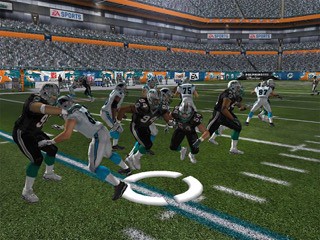A vibrant, small image seemingly from an unfamiliar computer game depicts a sports pitch populated by several players in black or grey uniforms, resembling American football attire. One player aggressively tackles another towards the left side of the pitch, which is lined with white markings. Cutting through the bottom of the image is a grey line intersected by a round circle composed of three segments, possibly part of the game interface or the pitch itself. The backdrop features a layered stadium crowd, vividly segmented into at least three distinct sections, with striking orange edges marking intervals between them. At the stadium's base, a series of multicolored signs encircles the perimeter, though they are too small to decipher. The overall scene is free of additional text overlays, focusing squarely on the dynamic sports action and the bustling ambiance of the crowd.